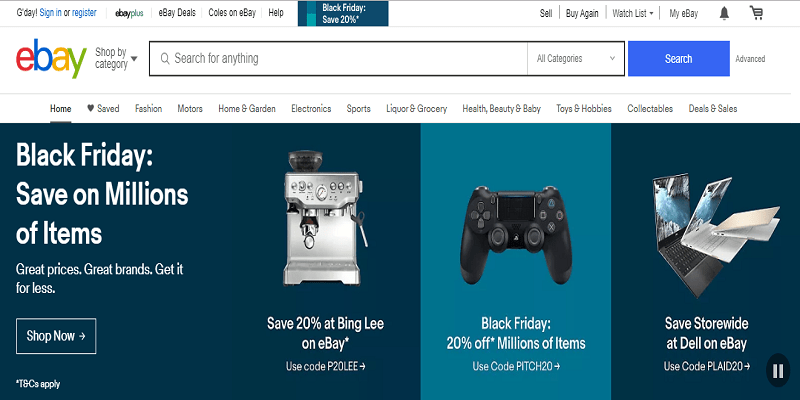The image showcases an eBay webpage, prominently featuring different sections and promotional banners. 

At the top, the page includes navigation options such as "eBay," "eBay Deals," "Codes on eBay," "Help," "Sale," "Buy Again," "Watchlist," and "My eBay," along with a special section for "eBay Plus." A search bar with a blue "Search" button and an "Advanced" search option is clearly visible.

Below the navigation menu, users can shop by category with options like "Home" (which is currently selected), "Save," "Fashion," "Motors," "Home and Garden," "Electronics," "Sports," "Liquor and Grocery," "Health, Beauty, and Baby," "Toys and Hobbies," "Collectibles," and "Deals and Sales."

The central portion of the webpage highlights a Black Friday sale banner, stating, "Black Friday: Save on millions of items, great prices, great brands, get it for less." A prominent "Shop Now" button with an arrow pointing to the right encourages users to take advantage of the deals.

Additional promotional banners offer various discounts, such as:
- "Save 20% at Bingley on eBay with code P20LEE," indicated with an arrow pointing to the right.
- "Black Friday: 20% off millions of items with code PITCH20," also indicated with an arrow pointing to the right.
- "Save Storewide at Dell on eBay: Use code PLAID20," accompanied by an arrow pointing to the right.